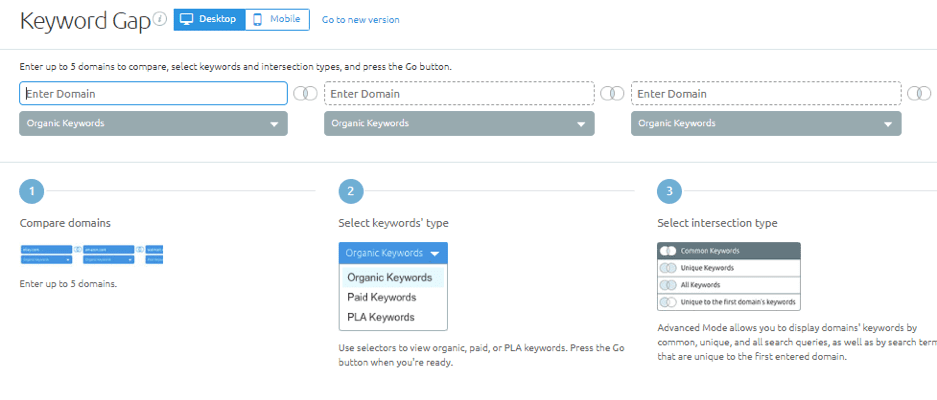The image is a left-to-right horizontal screenshot taken from a web page with a white background provided by the computer screen. At the top, in black text, it reads "Keyword Gap". Next to this heading, there is an option to select either "Desktop" or "Mobile," with "Desktop" highlighted in blue. To the right, there is a blue clickable text that says "Go to New Version." A thin gray line separates this section from the rest of the content below.

Below the line, another black text instruction reads, "Enter up to five domains to compare, select keywords and intersection types, and press the Go button." This is followed by input fields where domains can be entered. Each input field has a blue box around it, with gray dotted lines outlining the subsequent input fields. There are Venn diagram circles dividing each domain entry field. Beneath each "Enter Domain" field, "Organic Keywords" is written in gray with a clickable white arrow next to it.

Another gray line separates this section from the subsequent instructions marked by circles numbered one to three. Under circle number one, titled "Compare Domains," there are blue boxes with white text indicating "Enter up to five domains." Circle number two instructs to "Select Keyword Types," with clickable options for "Organic Keywords," "Paid Keywords," or "PLA Keywords." Circle number three is labeled "Select Intersection Type," with the "Common Keywords" option highlighted, among other selectable options.

The overall layout is meticulously designed to guide the user through the process of comparing domains, selecting keyword types, and choosing the intersection type for analysis.